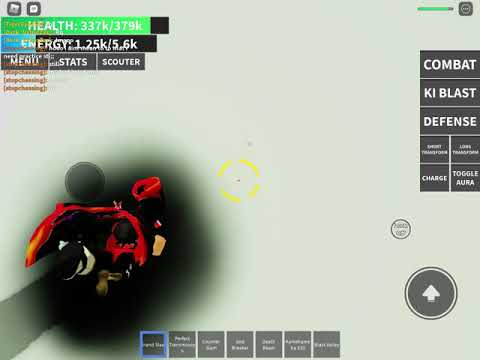This computer-generated image is a screen capture from a fighting video game, set against a predominantly white background. The top left corner features a green and black background displaying words in white font: "Health," "Energy," "Stats," "Menu," and "Scouter." The top right section similarly presents white text on a black background, listing "Combat," "KI Blast," "Defense," along with indistinct words like "Change," "Charge," and "Toggle Aura." 

In the bottom left corner, there is a confusing black blob with red splotches, possibly depicting an explosion or a character shot from the game. The bottom right corner includes a gray circle with an upward-pointing arrow. The bottom of the screen is lined with approximately eight gray boxes containing unreadable white text, with one box specifically outlined in blue.

Central to the image is a yellow target circle, which might represent a shooting lens or aim indicator. The right side of the screen features a darker gray segmented area with labels such as "Combat," "KI Blast," "Defense," "Charge," and "Toggle Aura." The overall layout and the combination of elements suggest an action-focused, possibly combat-oriented video game, likely played on a PC or console.